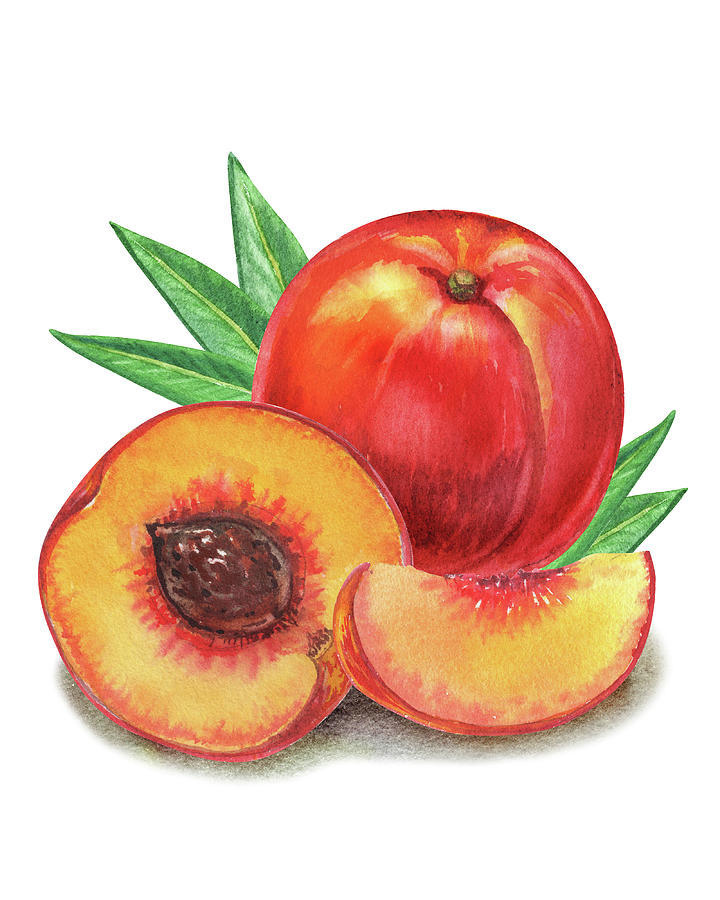The image features a detailed and realistic drawing or painting of peaches against a white background, likely rendered in colored pencil or watercolor. Central to the composition is a whole peach encircled by five vibrant green leaves. In the foreground, a peach is meticulously cut in half, revealing its orange flesh tinged with red hues and a prominently displayed pit. Adjacent to the halved peach is a separate, neatly sliced piece of peach with its pit removed, adding to the lifelike quality of the piece. The outer skin of the peach exhibits a striking blend of red and yellow tones, enhancing its realistic appearance. The artist has skillfully captured the intricate textures and colors, especially around the pit and the blush of the peach flesh.